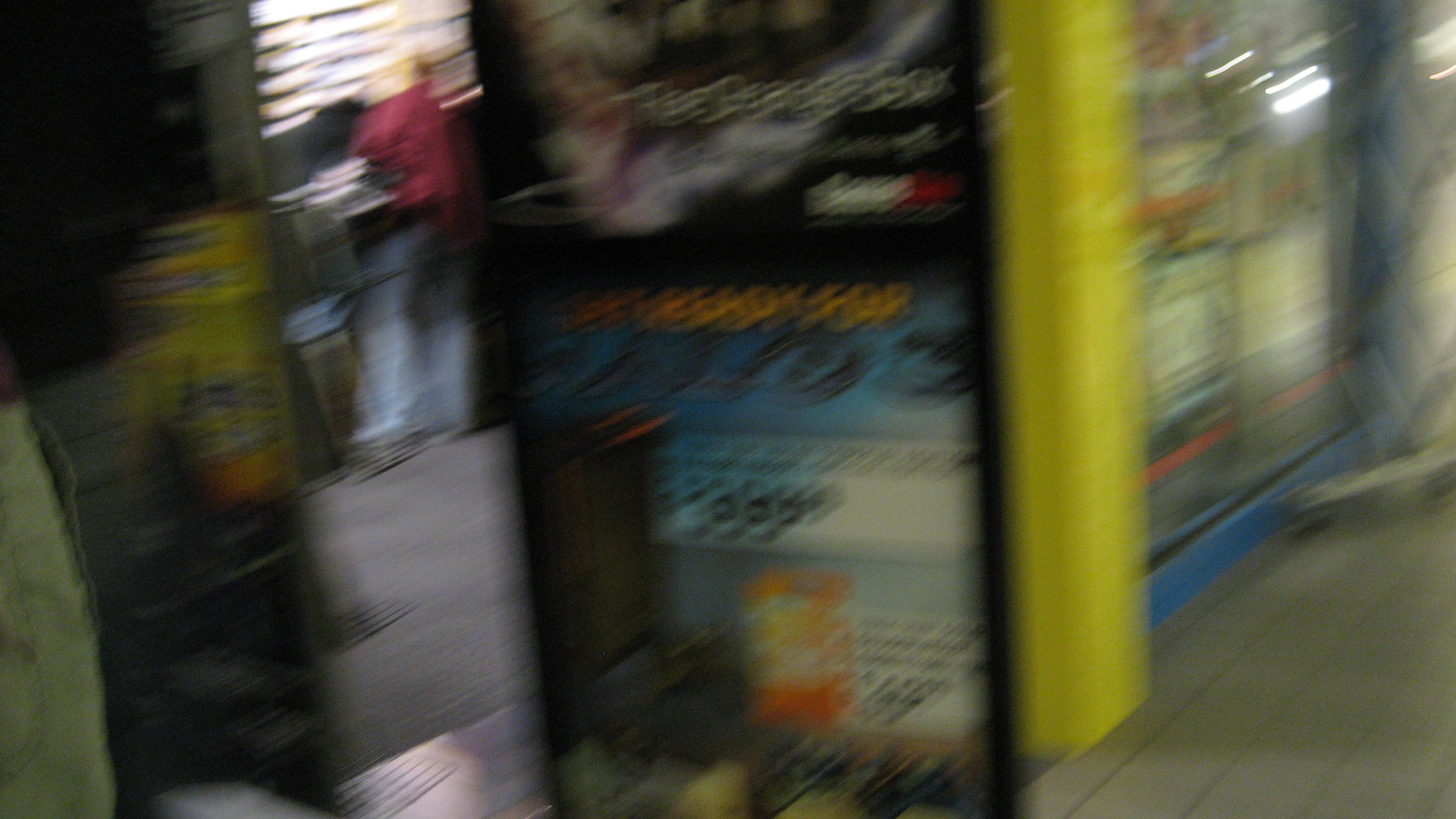The image is highly blurred and appears to have been taken with a moving camera, making the details difficult to discern clearly. The scene seems to depict the interior of what is likely a GameStop store, suggested by an advertisement that includes the GameStop logo. Above this logo, partially legible text appears to mention something like "dragon box," and below it, the phrase "ready for" can be faintly made out, followed by a price around $9.99. The advertisement also features an image that might be of a video game console.

On the right side of the image, there's a glass display case that seems to contain various boxes, perhaps holding merchandise or drinks, as it has the appearance of a cooler from a convenience store. Adjacent to this case is a floor-to-ceiling yellow pole or platform. To the left of this platform, there are multiple advertisements with a mix of dark and light colors, including blues, reds, and oranges, resembling typical retail posters with prices written in black text, although the exact products and prices are indiscernible due to the blurriness.

To the left, near the center of the shot, stands a customer in a red shirt and blue jeans, suggesting human activity within the store. In the background, shelves filled with merchandise can be faintly seen along with what appears to be a tiled floor, adding to the commercial atmosphere of the scene. Another yellow object, possibly another post or part of a display, is also barely visible.